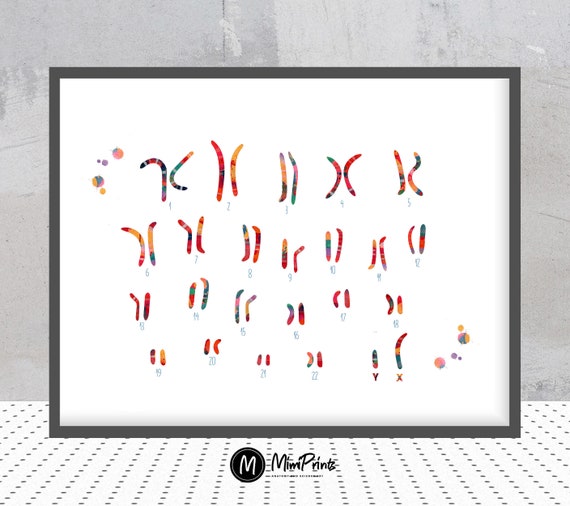The image depicts an art piece presented by MiniPrince, featuring a framed white canvas set against a light gray background and encased in a dark gray frame. The white interior of the frame holds 22 colorful, worm-like figures arranged in rows, each distinctly numbered from 1 to 22, along with an additional shorter figure labeled "X" and a longer one labeled "Y." These multicolored figures resemble chromosomes or candy-like objects, with hues of red, yellow, green, and more. The piece is accented with the word "Mimprints" in an italicized font enclosed within a black circle, adding a conceptual layer to the artwork. The entire composition leans slightly against the light gray wall, which appears to be covered with a pegboard, contributing a textured backdrop to the scientific or whimsical display.